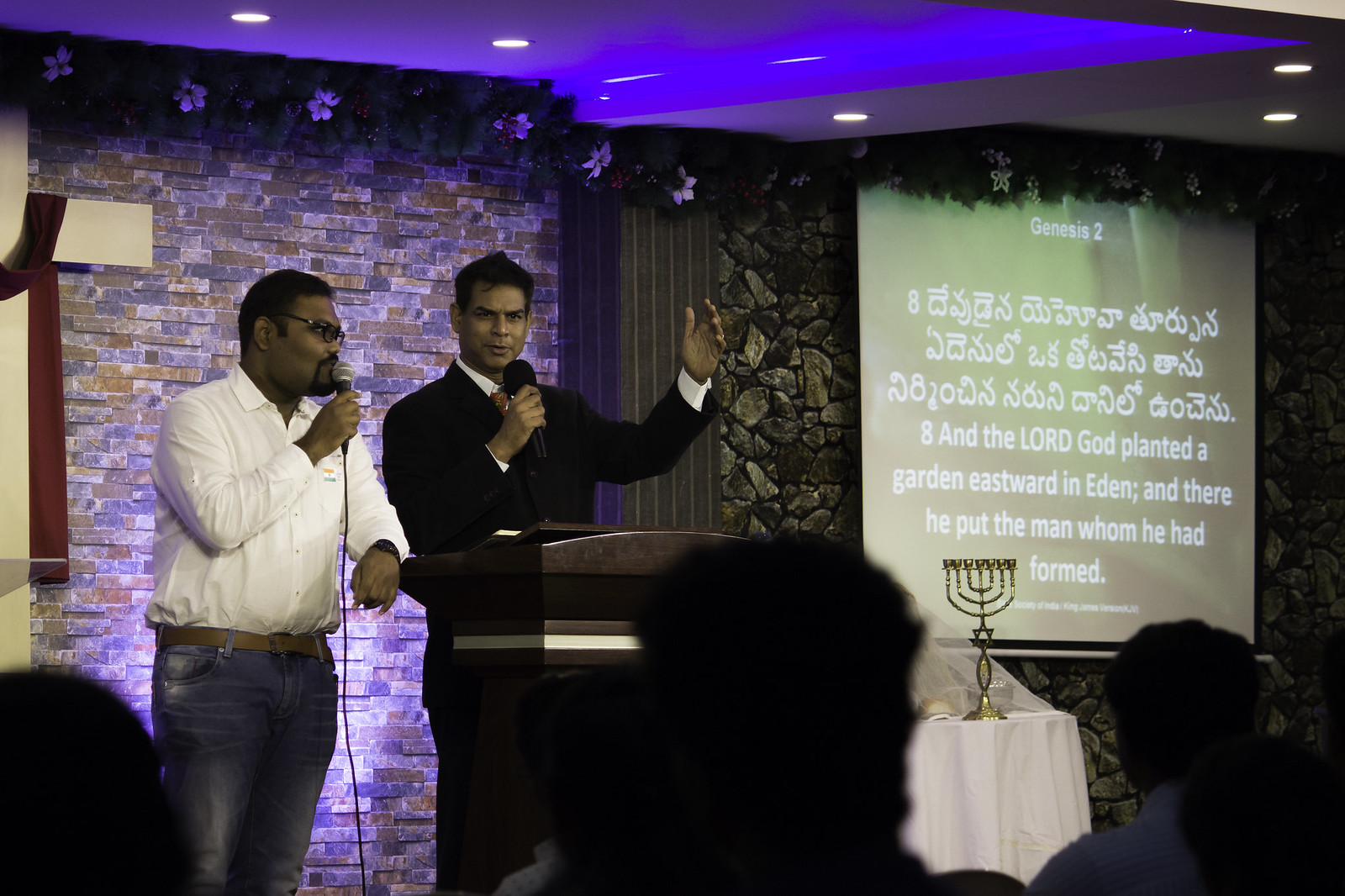In this dimly lit photograph resembling a nightclub but likely depicting a religious setting, two men are positioned just left of center behind a podium, engaged in speech with microphones before them. The man on the left, who appears to be African American, is dressed in a white shirt and somewhat faded blue jeans. The man on the right, who seems to be of Indian descent, is wearing a sharp black suit, red tie, and white shirt. To their right, a projector screen displays text from Genesis 2, in both English and possibly Hebrew or East Asian writing. The English passage reads, "and the Lord God planted a garden eastward in Eden, and there he put the man who he had formed." Below the screen sits a white table adorned with a menorah or candelabra. The background features a brick wall with rainbow-colored lighting, and the foreground is dotted with the silhouetted heads of audience members, further adding to the serene yet vibrant ambiance of the scene.